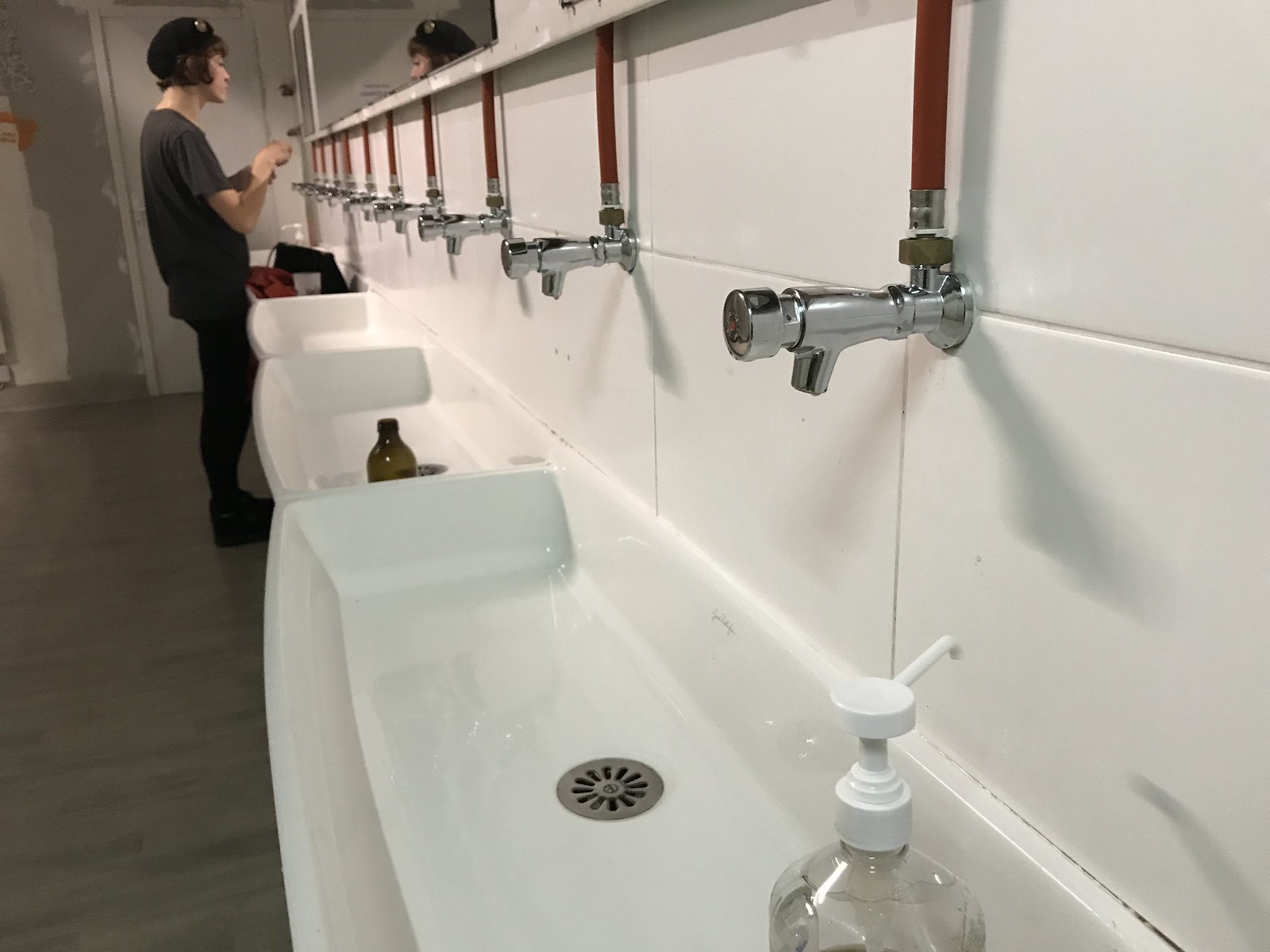The image captures a detailed scene of a communal public bathroom. The focus is on a series of white sinks, which are rectangular with slightly curved edges facing the user, and each features a silver, circular drain with a flower petal hole design. The faucets, which have push-button mechanisms, are wall-mounted and connect to visible red or dark red tubes that run behind rectangular mirrors, placed intermittently along the row of sinks. One soap dispenser made of white plastic is visible near the bottom center of the image, with ambiguity surrounding the presence of hand sanitizers. The floor is a very light brown, almost grayish, wood.

In the background, to the back left of the image, stands a woman wearing a gray t-shirt and tight black pants resembling leggings, paired with black footwear that could be either shoes or boots. She has short brown hair that curls slightly at the ends, reaching the top of her jawline. Additionally, she is wearing a hat resembling a beret, distinguished by a silver button. She is positioned in front of one of the sinks, with a white door also visible in the far back left of the image. The scene is well-lit, providing clarity to the details.